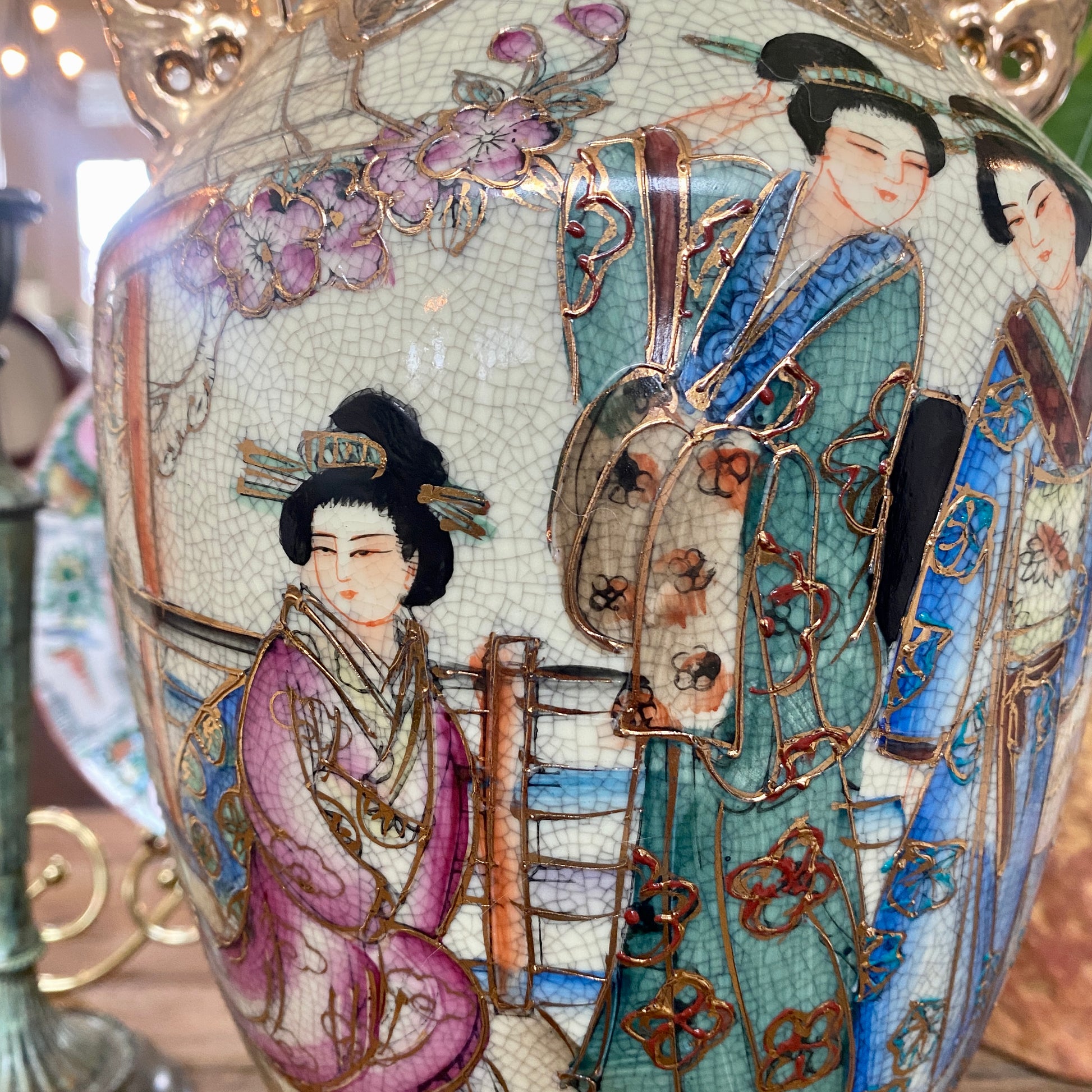This is a professional, close-up photograph of an exquisitely crafted oriental vase, possibly of Chinese or Japanese origin. The vase features three elegant women of Asian descent, intricately depicted in traditional attire. Each woman has her black hair styled in a bun and is adorned in vibrant, luxurious robes—the colors of which include purple, blue, and marine green or magenta. The women's garments are accentuated with flower designs and detailed with raised gold etchings, giving a tactile dimension to the visual art. The vase itself has a richly aged patina, hinting at its antique nature. Surrounding the figures are delicate pink flowers that extend towards the vase's top. The backdrop is slightly blurred, indicating an indoor setting, and the vase's brass elements shine with a polished luster, enhancing its refined appearance.